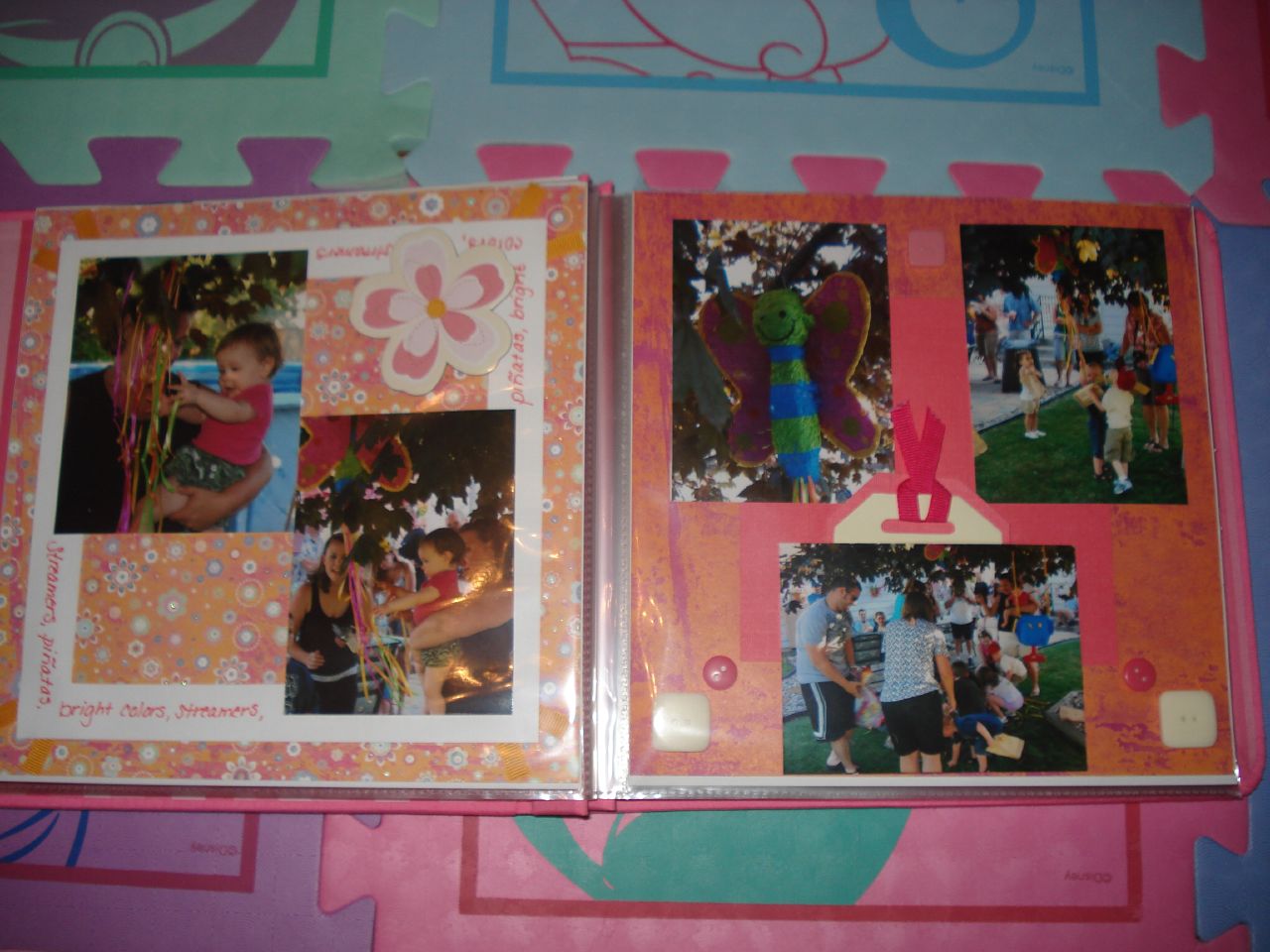The photograph depicts an open picture album set on a floor covered with large, interlocking foam puzzle mats, which are brightly colored in shades of light blue, light green, purple, and pink. A darker blue piece is partially visible on the right edge of the image. The album itself has a red cover and reveals two decorated pages. The left page features borders adorned with orange and various colored flowers. The top-left photo shows a baby being held, and another image below this depicts the baby, possibly playing with ribbons. The right page includes photos of toddlers with adults and captures moments from what appears to be a pinata event. The top-left image of this page shows a butterfly-shaped pinata that is green, blue, and purple. Adjacent images depict people swinging at the pinata and children collecting candy from the ground, suggesting the pinata has been broken. The entire setup combines to create a vibrant and nostalgic scene, ideal for preserving cherished memories.